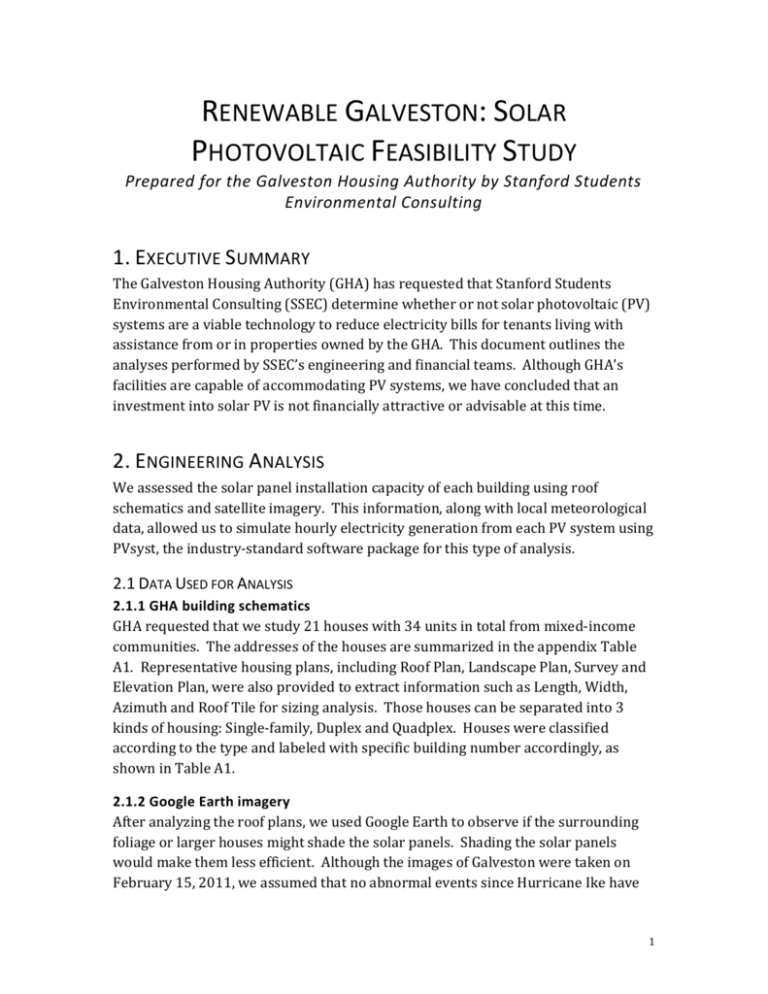This black-and-white photographic image features the front page of an article titled "Renewable Galveston: Solar Photovoltaic Feasibility Study." The document, prepared by Stanford Students Environmental Consulting for the Galveston Housing Authority (GHA), aims to assess the potential for using solar photovoltaic (PV) systems to reduce electricity costs for GHA tenants. The study is structured into various sections, with number one showing the Executive Summary. It highlights that although GHA's facilities can technically support PV systems, the financial analysis performed by SSEC indicates that investing in solar PV is currently neither financially attractive nor advisable. The document also features a number two, which marks the beginning of the Engineering Analysis section.